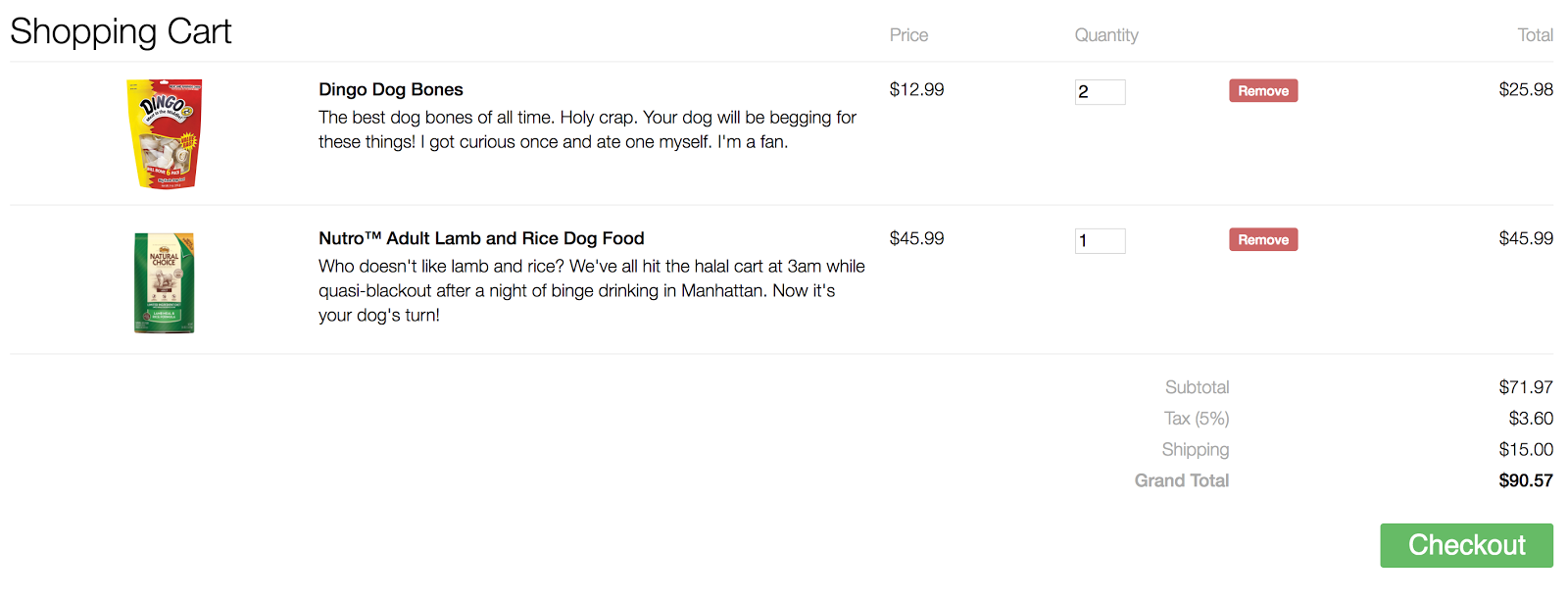Screenshot of a shopping app interface displaying the contents of a user's shopping cart. At the top of the screen, there are columns labeled "Item," "Price," "Quantity," and "Total," all written in black ink. Below these headings, two items are listed:

1. **Dingo Dog Bones**
   - **Packaging**: Small, with red and yellow colors and the word "Dingo."
   - **Description**: "Dingo dog bones, the best dog bones of all times, holy crap, your dog will be begging for those things. I got curious once and ate one myself, I'm a fan."
   - **Price**: $12.99
   - **Quantity**: 2
   - **Total**: $25.98
   - **Remove Button**: White text on a red background

2. **Neutral Alert Lamb and Rice Dog Food**
   - **Packaging**: Green with cream-white accents
   - **Description**: "Who doesn’t like lamb and rice? We’ve all hit the halal cart at 3 am while quite blacked out after a night of binge drinking in Manhattan. Now it's your dog's turn."
   - **Price**: $49.99
   - **Quantity**: 1
   - **Total**: $49.99
   - **Remove Button**: White text on a red background

At the bottom of the screenshot, the system calculates the overall costs:
- **Sub Total**
- **Tax (5%)**
- **Shipping**
- **Grand Total**: $90.57

A "Checkout" button is also visible, featuring white text on a green background. All other text on the screen is in black ink.